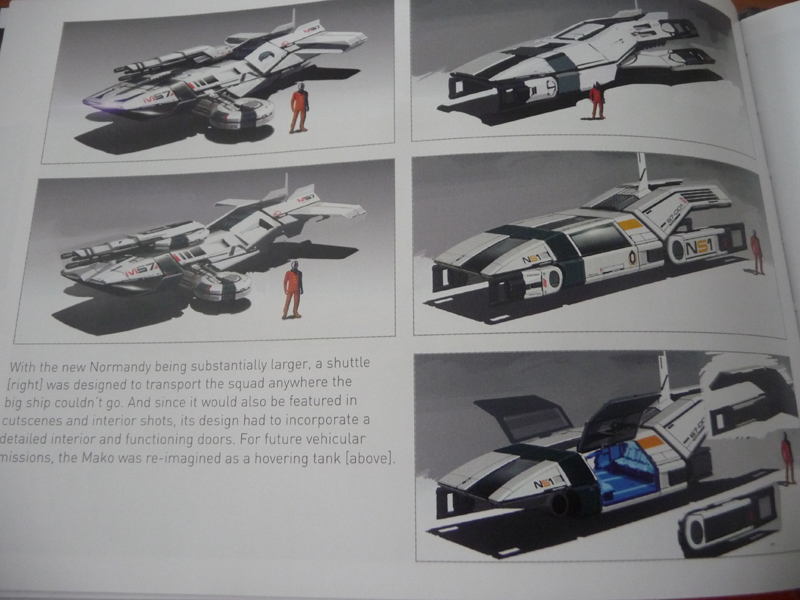This magazine page features a detailed exploration of a futuristic shuttle prop from a movie, showcased through five distinct images arranged in a series of panels. The left page of the book reveals the crease on the upper right side. At the top, there are two images of model airplanes with a graphic person standing in front of each one. Below, there are two more images of similar model airplanes, each accompanied by a person in a half-red, half-black uniform, with the one on the far right marked "N51." At the bottom, another image presents a side view of the plane. A descriptive blurb explains that with the new, significantly larger Normandy, a shuttle was created to transport the squad to locations inaccessible to the big ship. This shuttle design, featured in cutscenes and interior shots, required a detailed interior and functioning doors. Additionally, the Mako was redesigned as a hovering tank for future vehicular missions.